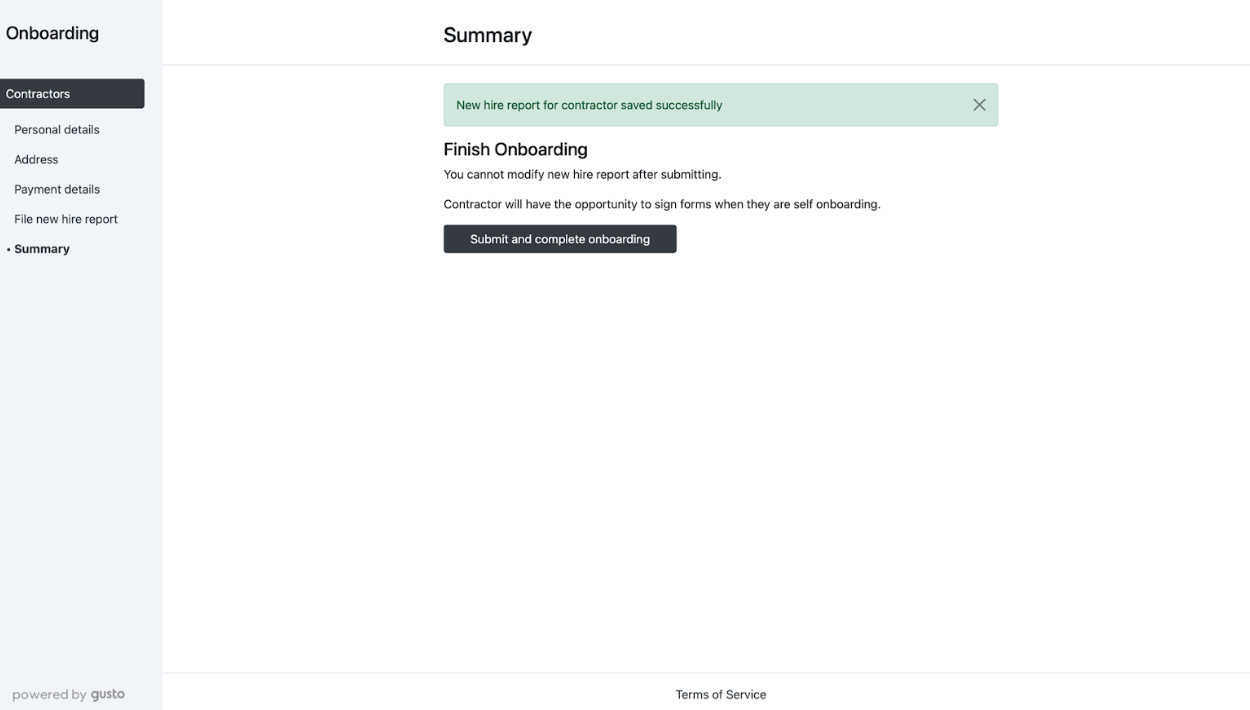The image displays a user interface related to onboarding contractors. 

On the far left, against a gray background, there's a bold black heading labeled "Onboarding." Below this heading is a black box with the word "Contractors." Underneath this box, there's a vertical list of items, which include "Personal Details," "Address," "Payment Details," "File New Hire Report," and "Summary."

On the right-hand side, the heading "Summary" is displayed. Directly below this is a green box with the following message: "No new hire report for contractors saved successfully." This green box also has an 'X' icon at the end.

Further down, the text reads: "Finish onboarding. You cannot modify new hire report after submitting. Contractor will have the opportunity to sign forms when they are self-onboarding." At the bottom, there's a black box with the text "Submit and Complete Onboarding."

Finally, the image includes a label at the base stating "Powered by Gusto."

This detailed caption should paint a comprehensive picture of the user interface for a reader.